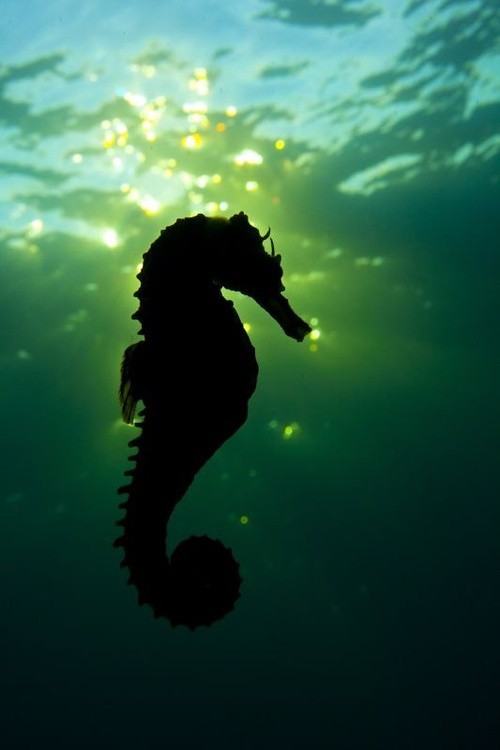This captivating photograph captures a seahorse in a vertical position beneath the ocean. Illuminated by rays of sunlight piercing through the ocean's surface, the water is a dazzling turquoise at the top, gradually transitioning to varying shades of green before finally melding into a deep, dark black-green at the bottom. The seahorse, portrayed as a striking black silhouette, stands out against this vibrant, ombre backdrop. Its tail is distinctively curled, with visible features that include a small fin and mouth. The sky behind the turquoise water suggests a bright, blue expanse, with the sun subtly peeking through and casting a mesmerizing glow underwater. Though the photograph lacks specific details about its origin, such as the exact location or the type of seahorse, it remains a stunning depiction of this marine creature in its natural habitat. The image is sized at 3 by 5 inches and contains no additional text or identifying information.